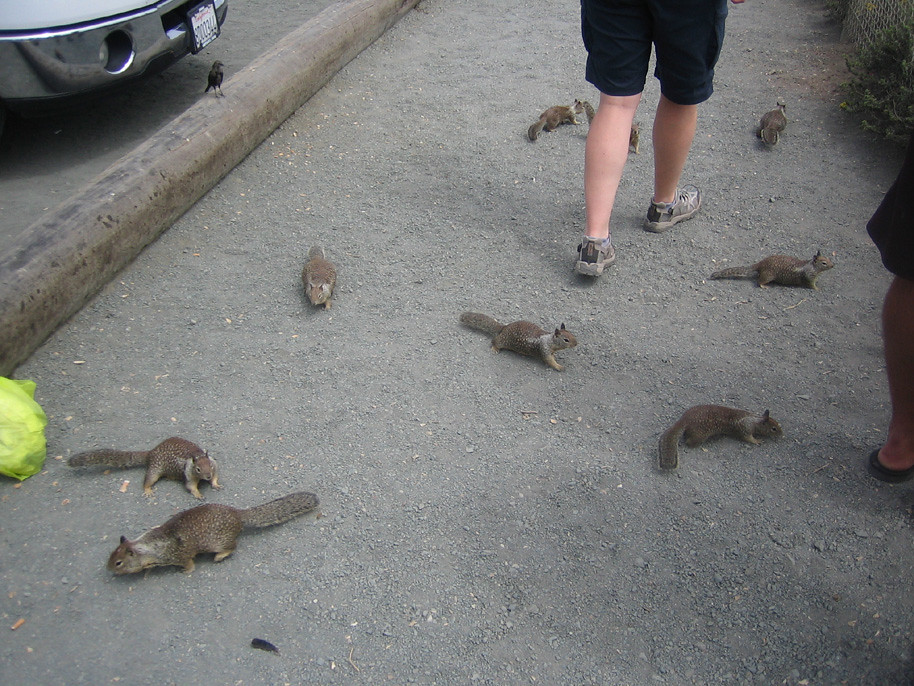This daytime, outdoor color photo captures a lively scene at the edge of a parking lot or on a gravel path. The foreground showcases a rough groundstone surface suitable for walking or biking. Prominently, there are nine gray squirrels scattered throughout the image, appearing very tame and accustomed to human presence, likely searching for food or handouts. The squirrels, each with bushy tails, are oriented in various directions, some pointing to the right and others to the lower left, spaced out as they scurry about.

In the upper left portion of the photo, the chrome front bumper of a car is visible, along with a license plate and wooden ties marking the parking spot. A log acts as a boundary for the parking area. Slightly to the right of center, we see the legs of an individual wearing dark athletic shorts and white sneakers. Another person is also visible further to the right, characterized by their black shorts and brown shoes. The lighting in the image is a bit dull, with no text or words present, creating a natural, candid atmosphere. Additionally, a green trash bag is noticed off to the left-hand side, and a bird is seen near the car, adding further detail to the bustling scene.